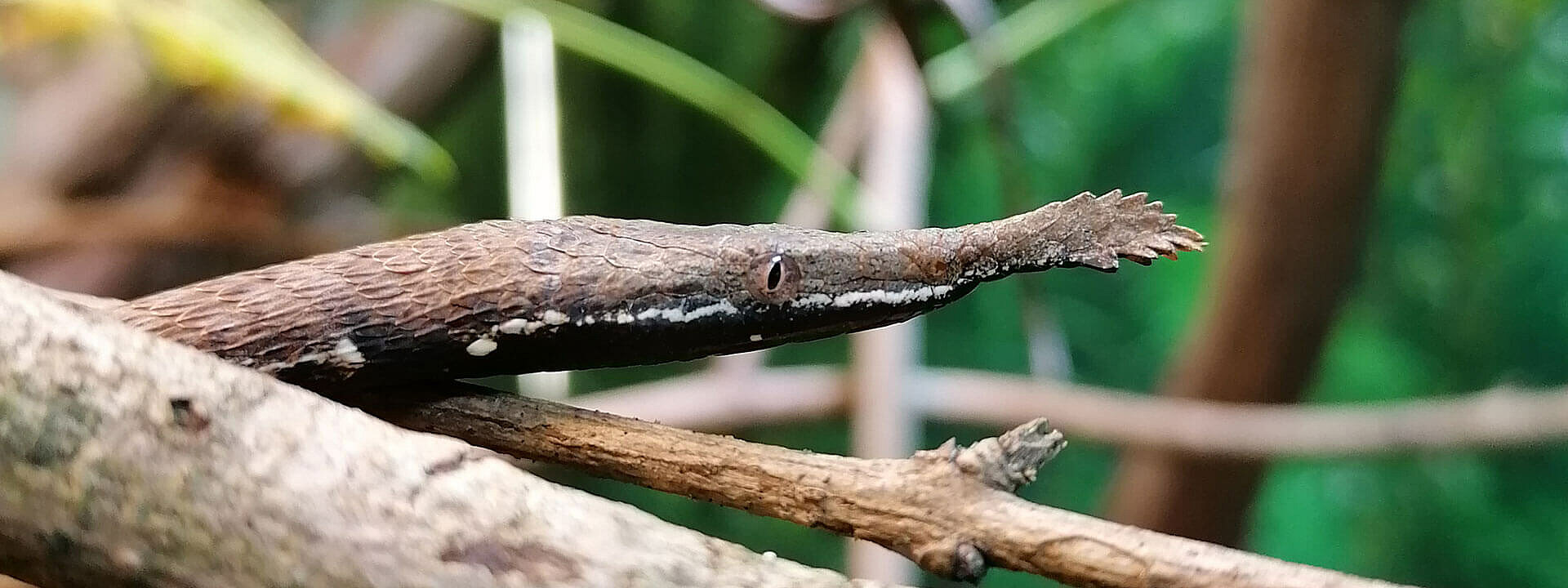In this highly detailed and close-up photograph, an exquisitely camouflaged reptile is displayed in what appears to be a forest or jungle setting. The creature, blending seamlessly with its surroundings, clings to a branch in the center of the image. It is a medium brown color with light tan and white chalky spots that mimic the texture and appearance of the twig it rests upon. Highlighting its remarkable camouflage, the reptile has a cylindrical, twig-like body and scales that match the brown tones of the branches around it. Its eyes are sharp and cat-like, giving it an eerie presence, with one eye subtly visible. The creature possesses an unusual nasal growth shaped like the top foliage of a pineapple, adding to its distinct appearance. The background is filled with green leaves and limbs, mostly out of focus, creating depth and emphasizing the creature's impressive ability to blend in with its natural habitat. The overall colors in the photograph are predominantly medium brown, light tan, and vibrant kelly green from the foliage.